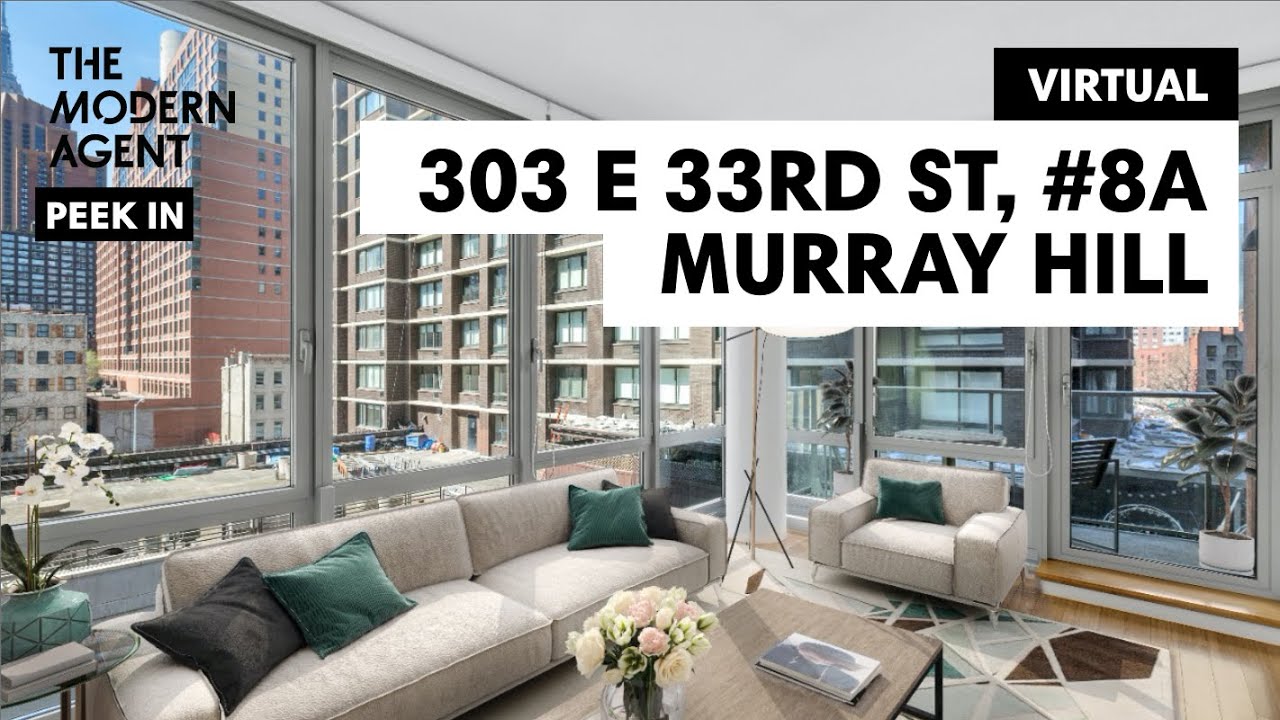This photograph showcases a modern living room with floor-to-ceiling windows that stretch along two walls, providing an expansive, panoramic view. In the upper left corner of the image, text reads "The Modern Agent." To the right, additional text states "Virtual Tour" followed by "303 East 33rd Street, Apartment 8A, Murray Hill."

The scene outside the windows is filled with numerous apartment buildings, each adorned with countless windows, contributing to a dense urban landscape. A blue sky with scattered clouds adds a touch of serenity to the cityscape.

The living room itself features a tan couch adorned with dark brown and dark green cushions, offering a cozy and stylish seating area. A green pot on the floor holds a beautiful white orchid, adding a touch of nature to the space. The brown coffee table complements the brown wooden floors, creating a warm and inviting atmosphere.

The patio outside invites one to step out and enjoy the views, while the red-brick buildings visible in the distance add to the classic New York City ambiance. Text elements in the photo use a mix of fonts and backgrounds: black font on a white background, white font on a black background, and "The Modern Agent" in black font without any background.

Overall, the photograph captures a sleek, modern living area with stunning urban views, beautifully blending interior comfort with the bustling energy of city life.